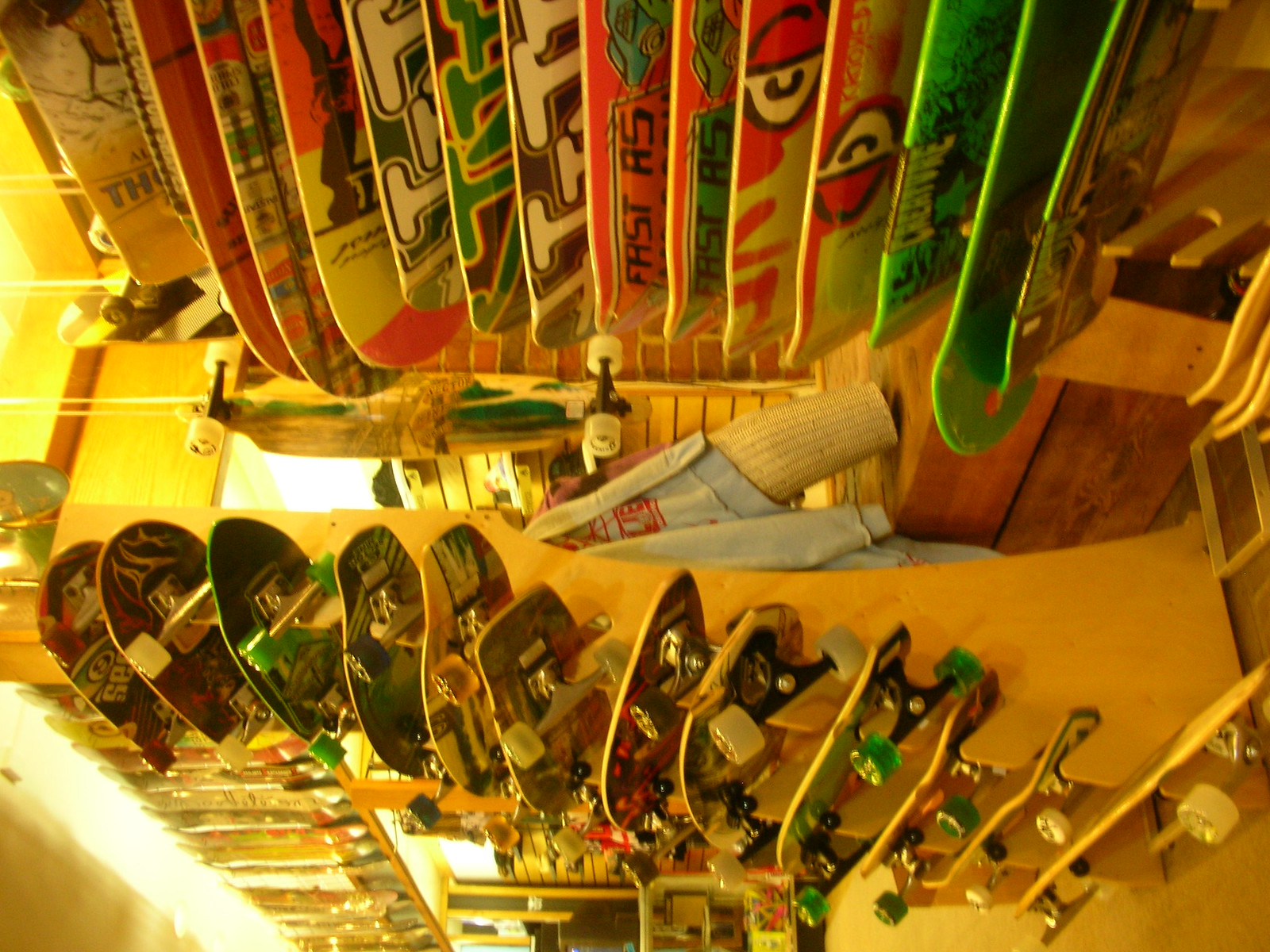This image, captured inside a skateboard store, has been rotated 45 degrees counterclockwise, making the scene appear sideways. A sepia-toned filter gives the photograph a nostalgic, yellowish hue. On what appears to be the left side of the rotated image, numerous skateboard decks are lined up, displaying a vibrant array of colors including green, pink, and white. These decks are stacked on a large wooden rack and do not have wheels attached. Towards the bottom of the image, which would be the lower left corner if correctly oriented, a variety of complete skateboards are visible, neatly arranged with their wheels on a tower-like display. The skateboards display an eclectic mix of designs and colors. In between these displays, a single shirt hangs prominently. The background features horizontal bricks and other skateboarding equipment, suggesting a well-stocked store environment lit by indoor lighting.